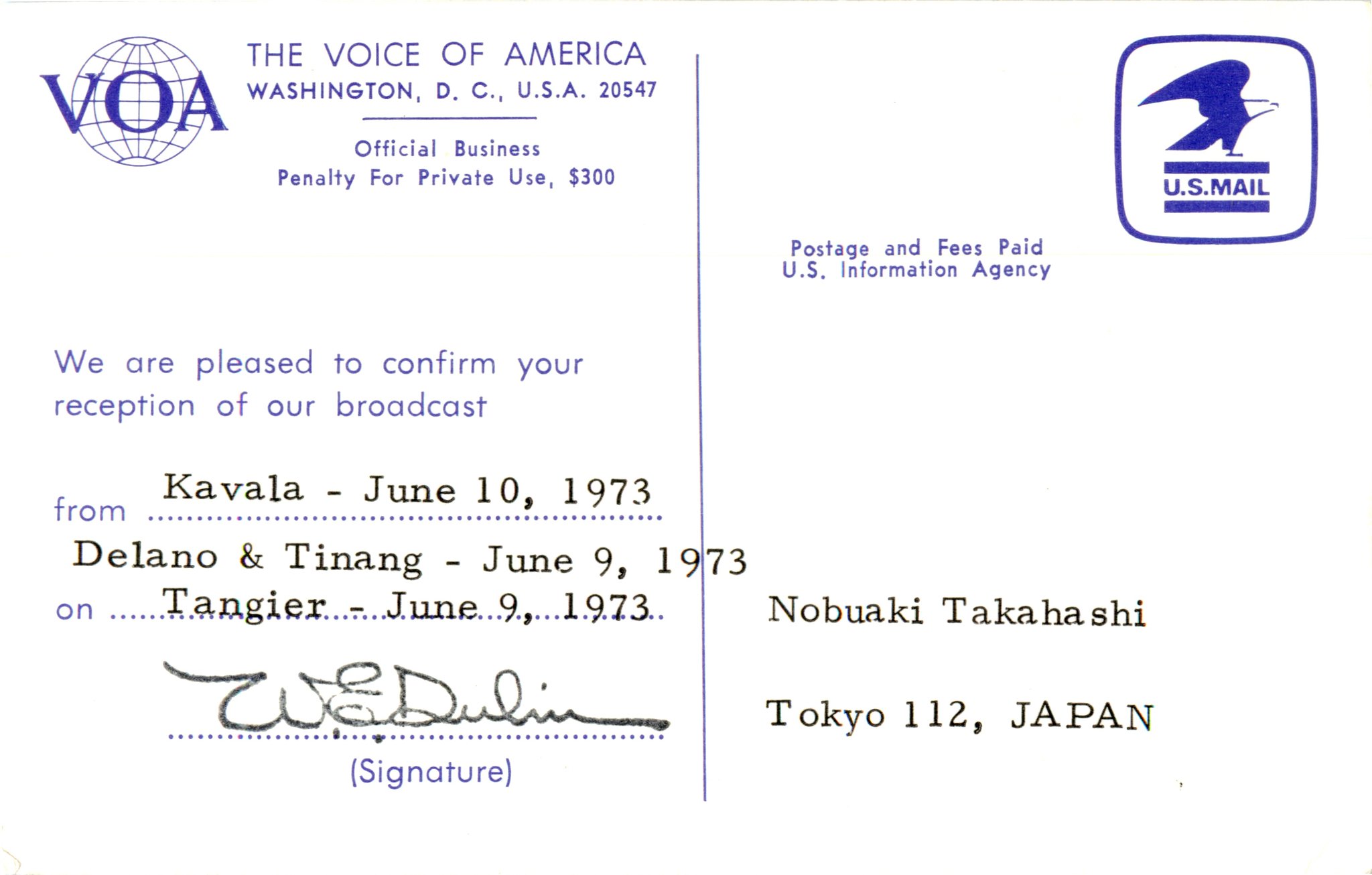This black-and-white postcard, printed in dark blue and oriented in landscape, serves as a confirmation of broadcast reception. The top left corner features the Voice of America (VOA) logo, a blue-outlined globe with the letters VOA superimposed on it, accompanied by the address Voice of America, Washington, D.C., USA 20547, and a disclaimer stating "official business, penalty for private use $300." In the top right corner is the U.S. Mail symbol with a bald eagle inside a blue square, next to the text "postage and fees paid U.S. Information Agency." Below, the postcard reads, "We are pleased to confirm your reception of our broadcast from Kavala, June 10, 1973; Delano and Tinang, June 9, 1973; and Tangier, June 9, 1973," followed by a signature. The addressee is Nobuaki Takahashi, Tokyo, Japan, with the address typed in a classic century black typeface.